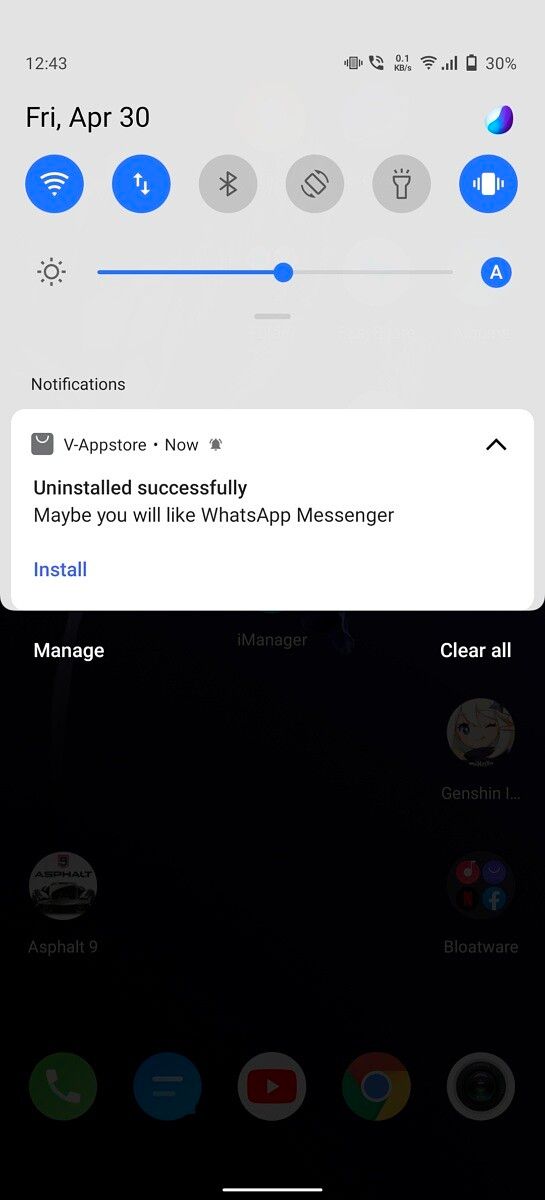In this image, we see what appears to be a screenshot of a mobile phone interface, identifiable by its tall rectangular shape. Starting at the top, there is a gray section occupying approximately the upper two-thirds of the screen. This section features the time "12:43" and a series of status icons on the right, including a signal bar, a phone icon, and a battery level indicator showing 30%. Immediately below the time, the date "Fri, April 30" is displayed.

Directly beneath the date, there is a row of icons representing various functionalities: Wi-Fi, data usage arrows, Bluetooth, screen rotation, flashlight, and an unidentified icon on the far right. Below these icons is a brightness slider.

The next section displays the word "Notifications" in bold. Immediately below, there is a white pop-up box proclaiming, "vStore app now uninstalled successfully. Maybe you will like WhatsApp Messenger, install." Just below this notification is a black box with white text offering two options: "Manage" and "Clear All."

Within this black box, there are icons for several applications. On the left, we have an icon for the mobile game "Genshin Impact," distinguished by a small anime character. Adjacent to it is an icon for "Asphalt 9," which features a racing car, suggesting it is a racing game. There is also a section labeled "Bloatware," containing application icons such as Netflix and Facebook.

Towards the bottom of the screen, we see the home row of navigation buttons typical of many smartphones: the phone key, messaging key, YouTube, Google Chrome, and a camera icon.